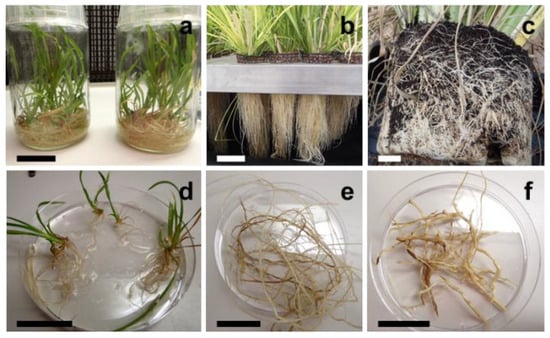This image depicts a series of six square-shaped photos arranged in two rows, three per row, illustrating the growth cycle of small plants. Each picture is labeled with a corresponding letter from A to F, starting from the top left. 

- **Image A:** Shows two clear, see-through containers partially filled with light tan soil. Emerging from the soil are small, green plants with long, blade-like leaves. The containers' transparency allows for a clear view of the curling roots at the bottom.
  
- **Image B:** Features the same containers now situated on a white tray, likely with the containers removed or opened. The plants have grown taller, with their leaves transitioning from a soft, darker green to a stiffer, lighter green. Thick roots extend downward below the containers, indicating a hydroponic growth stage.
  
- **Image C:** Provides a close-up, top-down view of the dense, white roots entangled in the dark soil.

- **Image D:** Shows some plants that appear to have been transferred to a petri dish. These small plants, possibly baby ones, are immersed in water, with their roots splaying out in various directions. The leaves maintain their green, blade-like appearance.

- **Image E:** Focuses on the roots alone, with the plants removed, revealing an intricate network of roots occupying the dish.

- **Image F:** Depicts the dish now emptied of water, with the roots appearing dried and somewhat shriveled.

This comprehensive visual timeline captures the plants' progression from initial growth in soil through stages of hydroponic development, to eventual root isolation and drying.